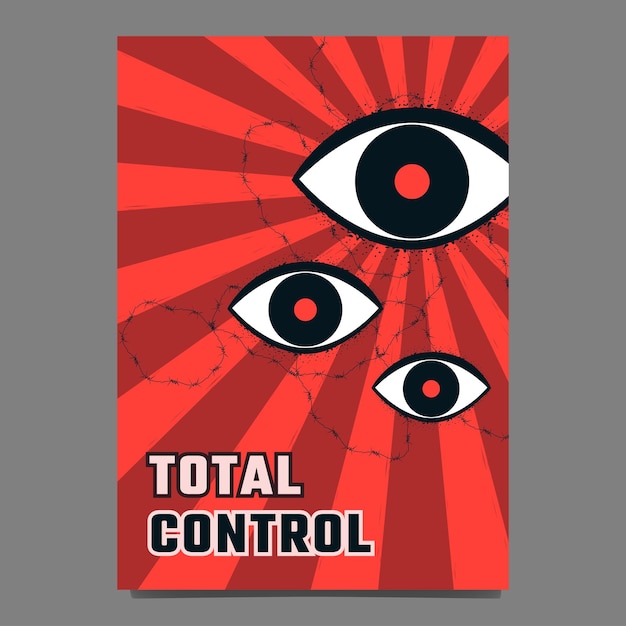The image in question is a striking poster set against a radiant red background, which emanates rays from the largest of three black-rimmed eyes positioned diagonally from the top right corner. Each uniform eye features a white cornea and a black pupil with a red dot in the center, perfectly matching the lighter of the two shades of red used for the radiating rays. The sizes of the eyes descend from large to medium to small. Adding to the intense, watchful feel of the piece, these eyes are visually bound together by a chain-link fence effect, suggesting entrapment or surveillance. At the bottom left corner of the poster, the bold phrase "TOTAL CONTROL" is prominently displayed, with "TOTAL" in white letters outlined in black, and "CONTROL" in black letters outlined in white. This graphic, devoid of any artist or author attribution, compellingly conveys themes of control and monitoring, reminiscent of conspiracy theories wherein every move is watched.